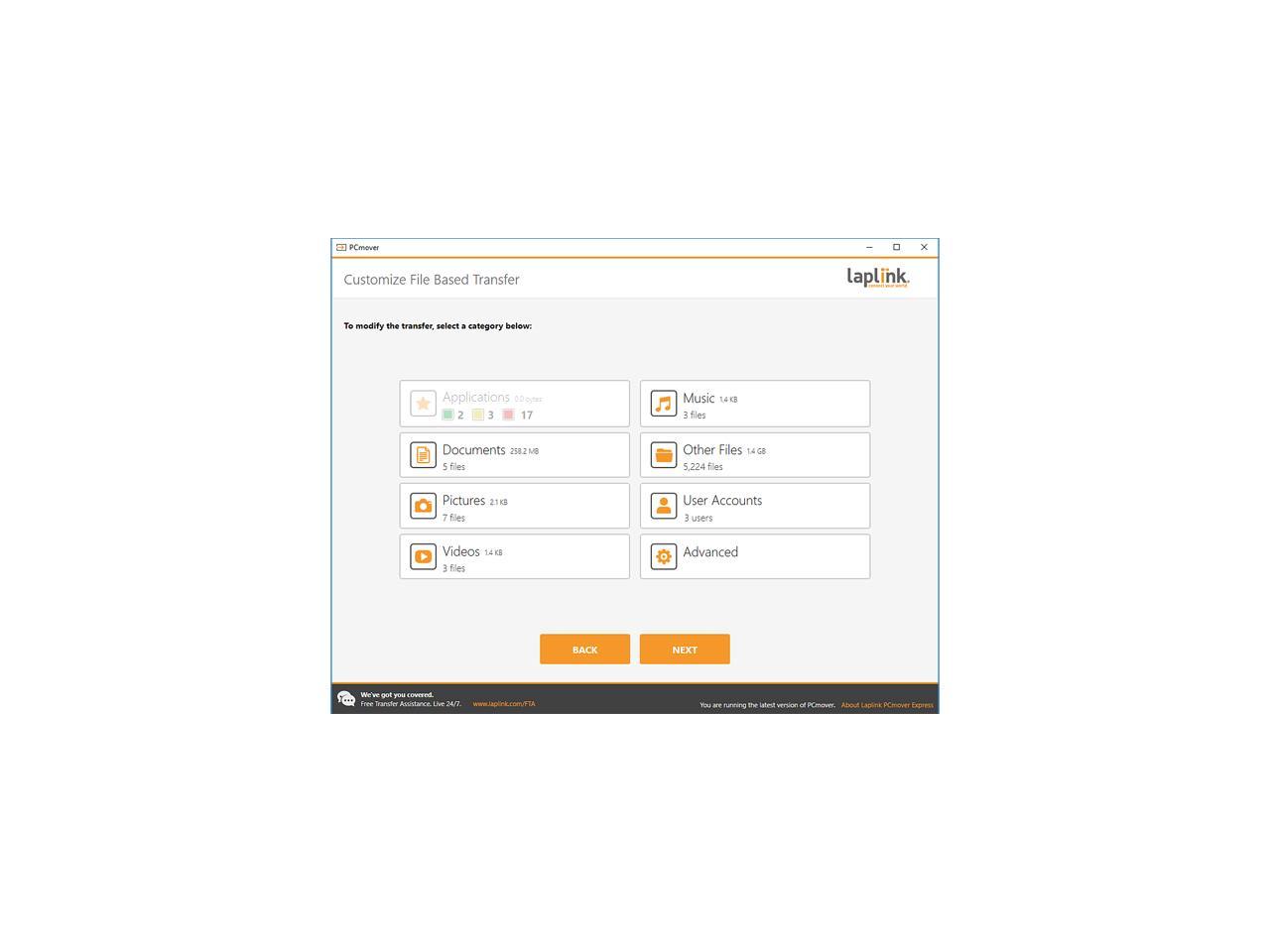This is a detailed and cleaned-up caption:

The image depicts a small section of a primarily gray-toned web page, accented with yellow and orange elements, accompanied by some black detailing. At the top center, there's an indistinct yellow logo with text to its right, potentially indicating "PC Connect." Towards the right side of the header, there are minimize, maximize, and close buttons. "Customize File Based Transfer" is written at the uppermost part of the page in gray font. To the right of this, the word "Laplink" is displayed with "Lap" in gray and the "i" in "link" highlighted in yellow. Below this header, there's an instruction that reads, "To modify the transfer, select a category below." The interface includes several rectangular buttons labeled "Applications," "Documents," "Pictures," "Videos," "Music," "Other Files," "User Accounts," and "Advanced." Two prominent orange buttons labeled "Back" and "Next" are located at the bottom of the page, over a black banner.